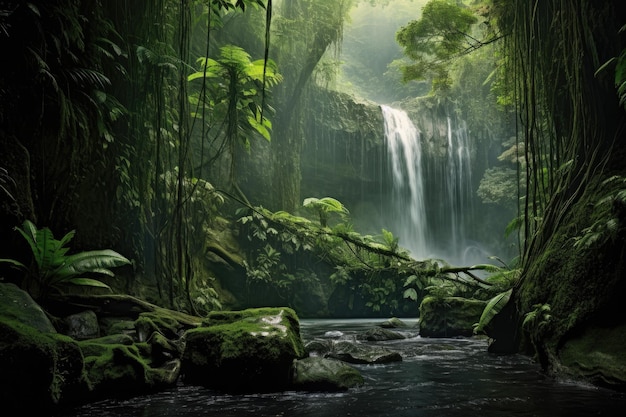The image depicts a lush, vibrant forest scene that may be either a photograph or a digitally generated illustration. Dominating the center is a striking white waterfall with a subtle greyish tinge, cascading down into a dark body of water that appears either as a creek or part of a small lake. The entire landscape is bathed in greenery, from the verdant ferns, bushes, and various plants with green leaves, to the dark green or brown hanging vines. Moss-covered rocks add texture and depth to the natural setting. Above the waterfall, sunlight illuminates an open area, creating a contrast with the otherwise dense forest, which is populated with trees, shrubs, and additional plant life. The overall composition of the rectangular image emphasizes the serene and untouched beauty of the wilderness.